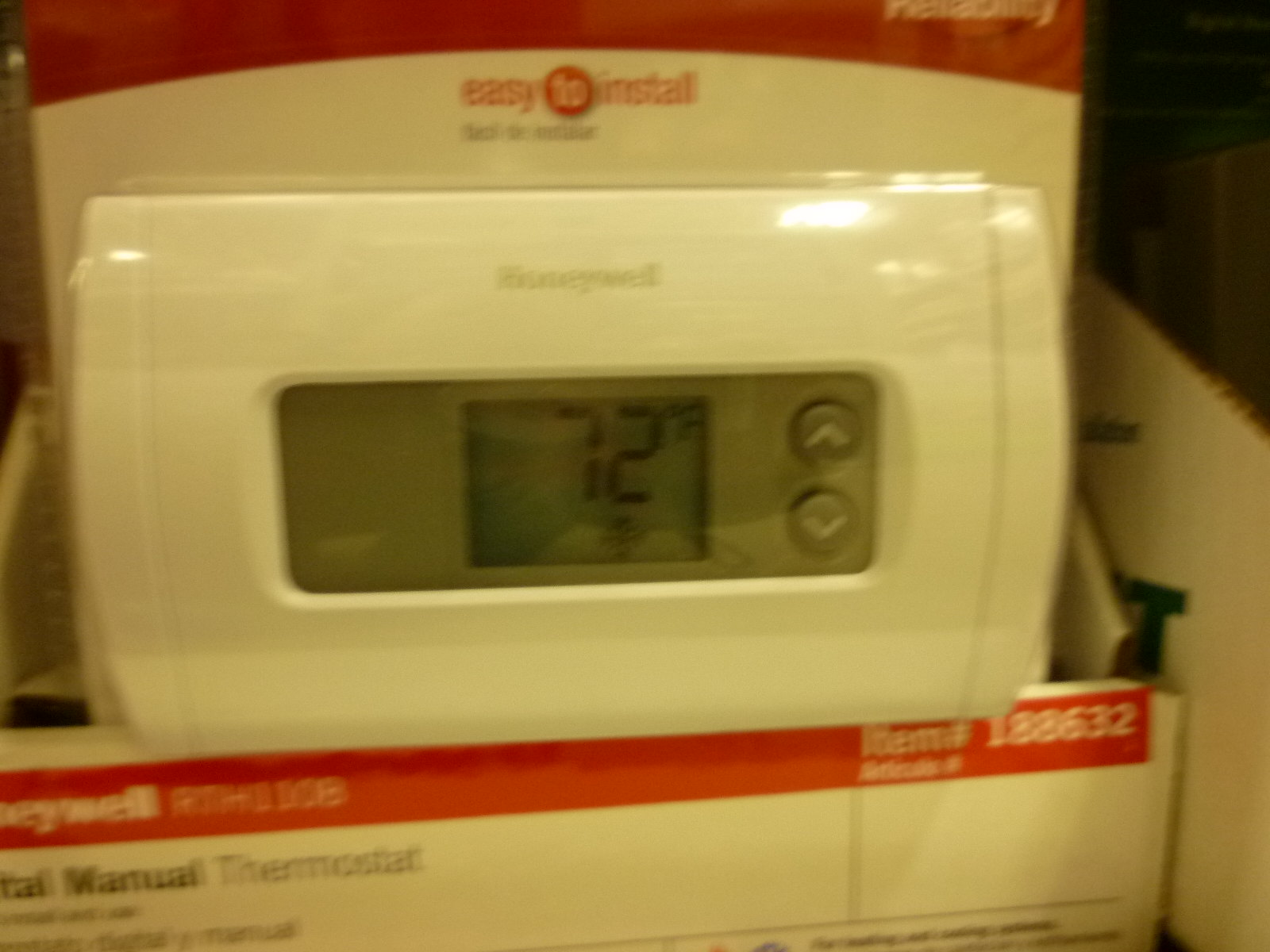The image showcases a Honeywell thermostat, still encased in its plastic packaging, positioned within its original box. The photograph is slightly blurry but provides sufficient detail. At the top of the image, a red banner is visible, followed by a white banner with bold red text that reads "Easy to Install." The thermostat itself is rectangular and white, prominently branded with the Honeywell logo at its center.

A rectangular display window on the thermostat shows a smaller square area indicating the temperature, set at 72 degrees Fahrenheit. To the right of this display are two circular buttons, marked with up and down arrows for temperature adjustment. 

The packaging is designed with a white base and a red stripe at the top, also bearing the Honeywell name. Below this, the item number "188632" is listed. Towards the bottom of the box, partially cut-off text suggests it is a manual thermostat. Positioned in the far right corner of the image is an adjacent cardboard box.